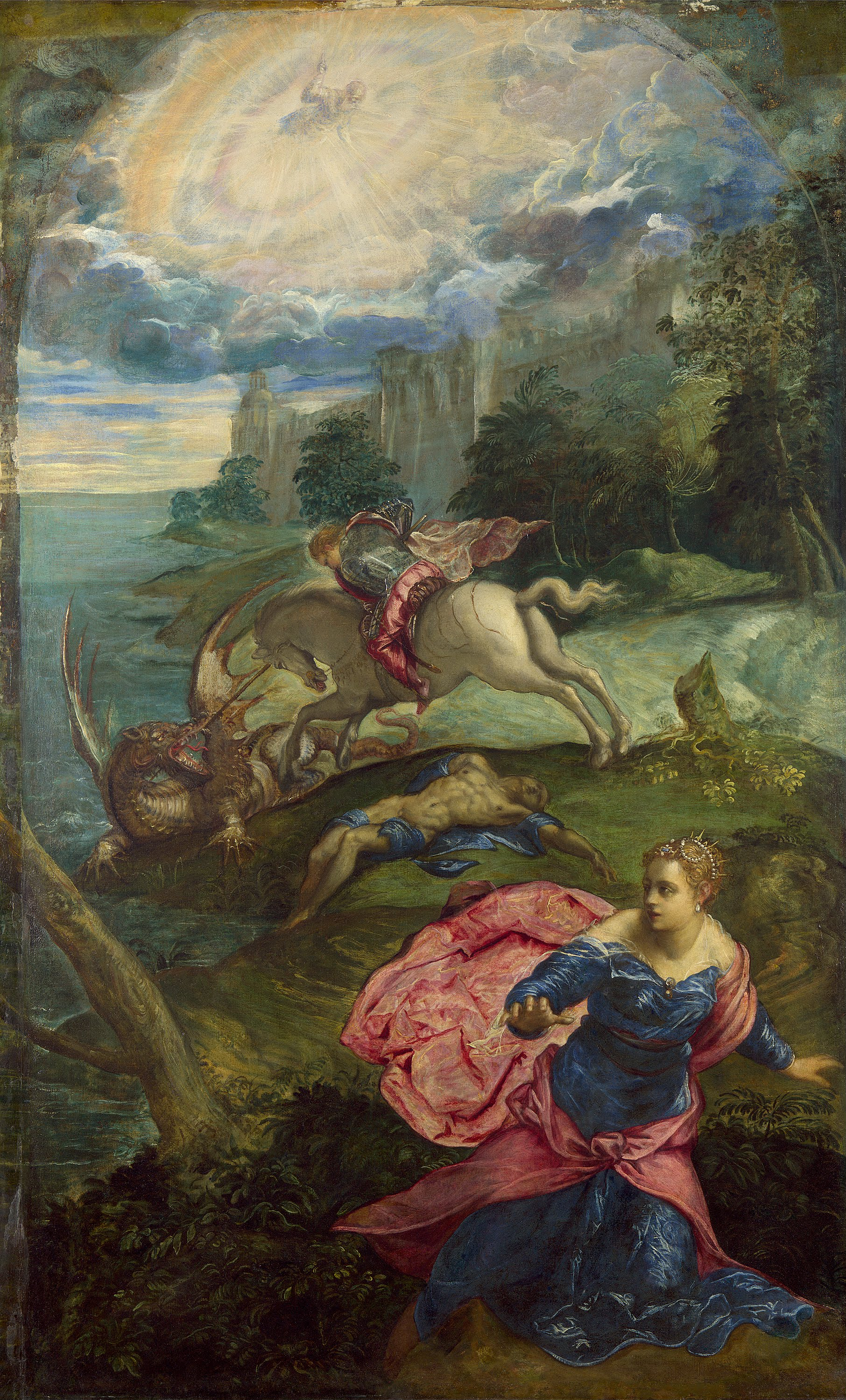This vibrant Renaissance oil painting by Tintoretti, titled "Saint George and the Dragon," is a masterful depiction of a mythological scene filled with dynamic elements and rich details. Set against a lush, dark green forest with verdant grass and towering trees, the painting immerses the viewer in a fantastical world. In the bottom right corner stands a blonde woman, dressed in a long blue gown adorned with a pink silk shawl draped around her neck, who appears to be fleeing toward the right side of the image. Her gaze is cast back over her right shoulder, conveying a sense of urgency and fear. Just behind her, a heroic figure, Saint George, charges forward on his majestic white horse. He is poised to battle a ferocious dragon that emerges from the aqua-colored ocean. 

The dragon and Saint George's steadfast steed are locked in a fierce confrontation, with the dragon baring its teeth in a display of aggression. Behind this intense struggle, a mystical, partially submerged castle extends into the water, adding to the painting's enchanting atmosphere. The sky above is a swirl of ethereal, gray clouds with a radiant, golden sun breaking through. At the heart of this celestial display, a divine figure with an aura is seen, raising a hand as if to chastise or intervene in the ongoing battle between Saint George and the dragon. This divine presence adds a layer of sacred drama to the scene. The painting, rendered in a style of abstract surrealism typical of the Renaissance period, is not only a feast for the eyes but also a vivid storytelling canvas that captures an epic clash between heroic valor and mythical terror.